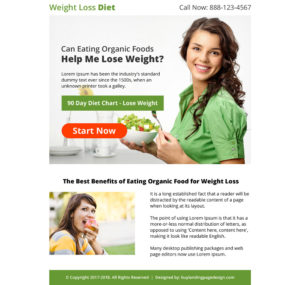Screenshot of a website featuring information on weight loss through diet. At the top, the heading reads "Weight Loss Diet" followed by a call-to-action "Call now: 888-123-4567". Below this, a photograph shows a young, fair-skinned woman with long, wavy dark hair, smiling at the camera. She is dressed in a short-sleeved green blouse and is holding a fork in her left hand and a white bowl of salad in her right hand.

On the left side of the screenshot, the text "Can Eating Organic Foods Help Me Lose Weight?" is visible. The subsequent text is blurred and unreadable. Beneath this, a green rectangle contains the text "90 Day Diet Chart, Lose Weight", and below that, a red oblong button says "Start Now".

Further down, another photograph shows a different young, fair-skinned woman facing the camera with a big smile. She has long, dark hair and wears a gray and yellow striped sweater. She is holding a piece of fruit in her left hand, preparing to take a bite. The text "The Best Benefits of Eating Organic Food for Weight Loss" is displayed next to her, followed by more blurry, unreadable text.

At the very bottom of the image, a green border contains additional text that is too small to be legible.